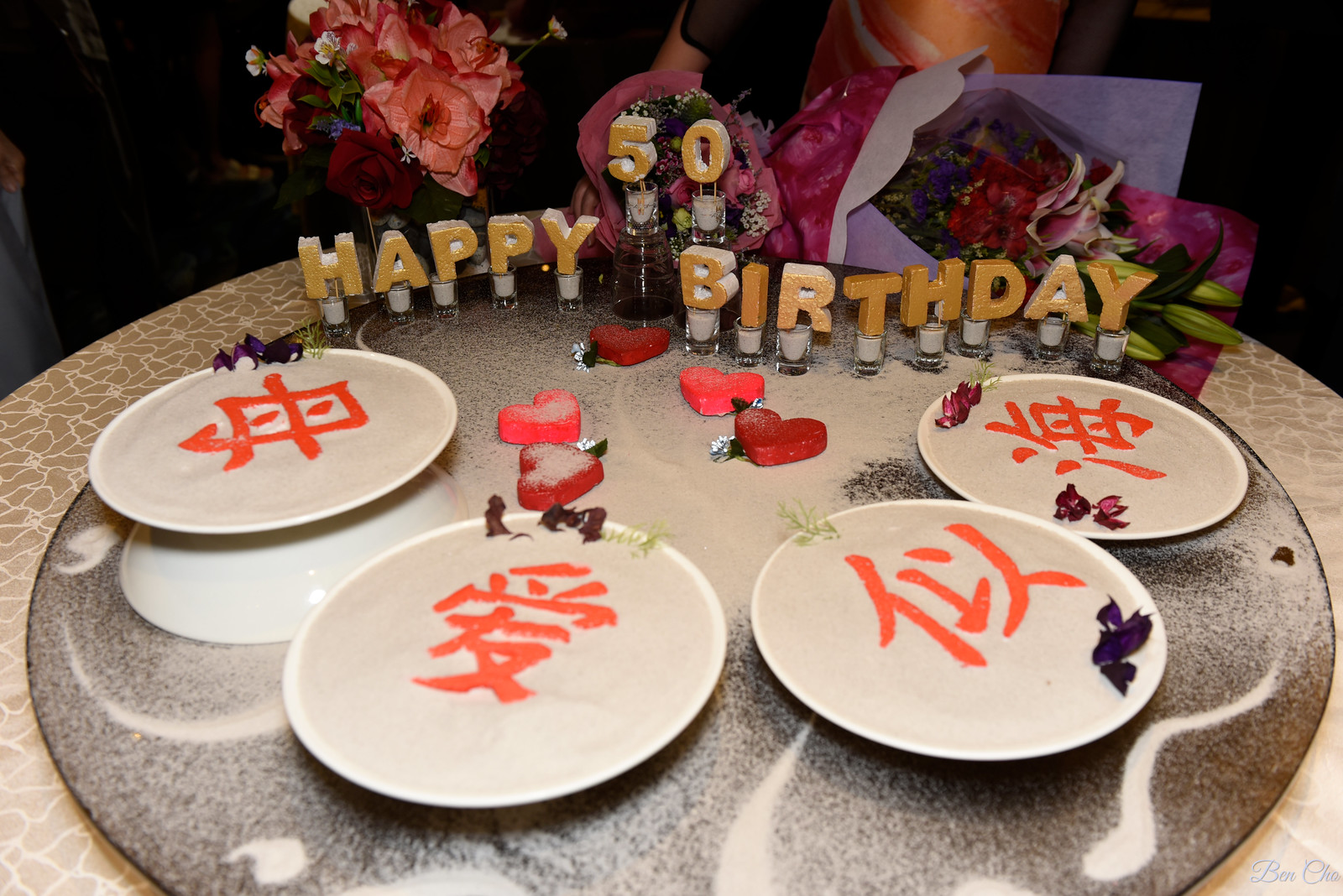On the table, there is a circular disc with white streaks and a dusty brown finish. The table surface is an intricate mosaic of misshapen tiles. In the background, candles are lined up, each adorned with a letter and number, with the most prominent being the number "50" elevated above the rest. Below these candles, starting from the left, are candles that spell out "Happy Birthday." In front of the candles, five heart-shaped cutouts, embellished with white sprinkles, are meticulously arranged. 

Plates are positioned in a semicircle formation from the upper left side to the lower right. These plates are white on the outside with a light cream-colored interior. Each plate features an orange foreign language character and contains what appears to be a soup, garnished with purple leaves and a touch of green.

The background is dominated by an array of purple and pink flowers, set against a predominantly dark backdrop. On the right side, there is a cover for the flowers made from a sheet of purple paper.